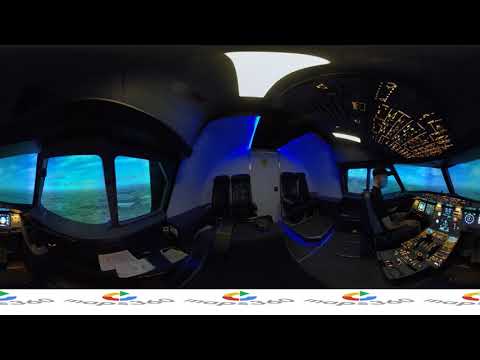The image is a color panoramic photograph of a futuristic aircraft cockpit, presented in landscape orientation. It appears to combine three photographs seamlessly into a cohesive panoramic view. The left section of the image showcases a view from inside the cockpit through three segmented windows, akin to those found in an airplane or bus, with some papers visible in the foreground. 

The central section draws attention to the detailed interior of the cockpit, focusing on a central passage with a round circular structure at the end. This structure features a white door flanked by four black seats on either side, with blue lights illuminating the scene. The cockpit panels are dark gray with a blue hue emanating from some instruments.

On the right side, the focus shifts to a pilot seated in the cockpit, surrounded by a plethora of lit-up controls and instrument panels both in front and overhead. The pilot sits on the right-hand side, and the area behind him includes three tall chairs and a white section adjacent to three windows. The background features multi-colored lights and indicators, characteristic of a high-tech, possibly video game-inspired setting. At the forefront, there is a visible strip with panoramic filter information and an arrow.

Overall, the image combines elements of representationalism with a futuristic touch, capturing the intricate details of an advanced cockpit environment.